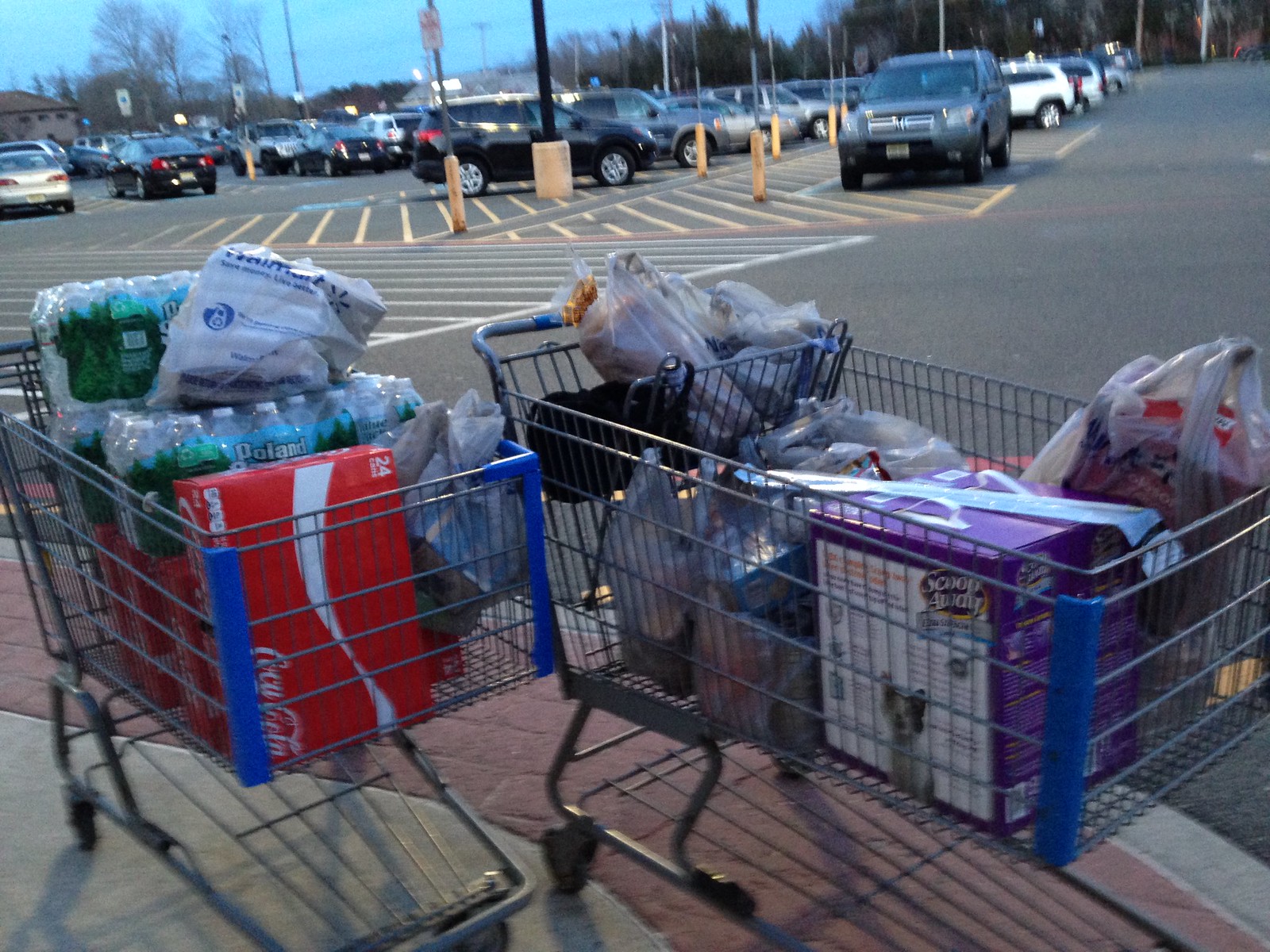The photograph captures two fully loaded shopping carts angled towards the bottom right, situated on a sidewalk with a red brick streak and plain concrete. The shopping carts take up the bottom half of the image and stand prominently against the backdrop of a busy parking lot filled with several rows of cars. The scene is enveloped in the dim light of dusk, casting a darkish hue over the area, with street lights beginning to illuminate the sky, which is an aqua blue color, along with the silhouettes of trees lining the horizon.

The left shopping cart is brimming with items, most noticeably featuring multiple red cases of Coca-Cola cans and three cases of bottled water, presumably by Poland Spring, though the brand is unclear. A few Walmart plastic bags are also visible, suggesting the origin of the purchase. On the right, the shopping cart contains a variety of items, including a prominent purple box labeled Scoop Away kitty litter. This cart also has several plastic Walmart shopping bags filled with groceries, and a black purse is nestled in the front section of the cart. The entire scene exudes the bustling activity of a shopping trip nearing its end as the day transitions into night.